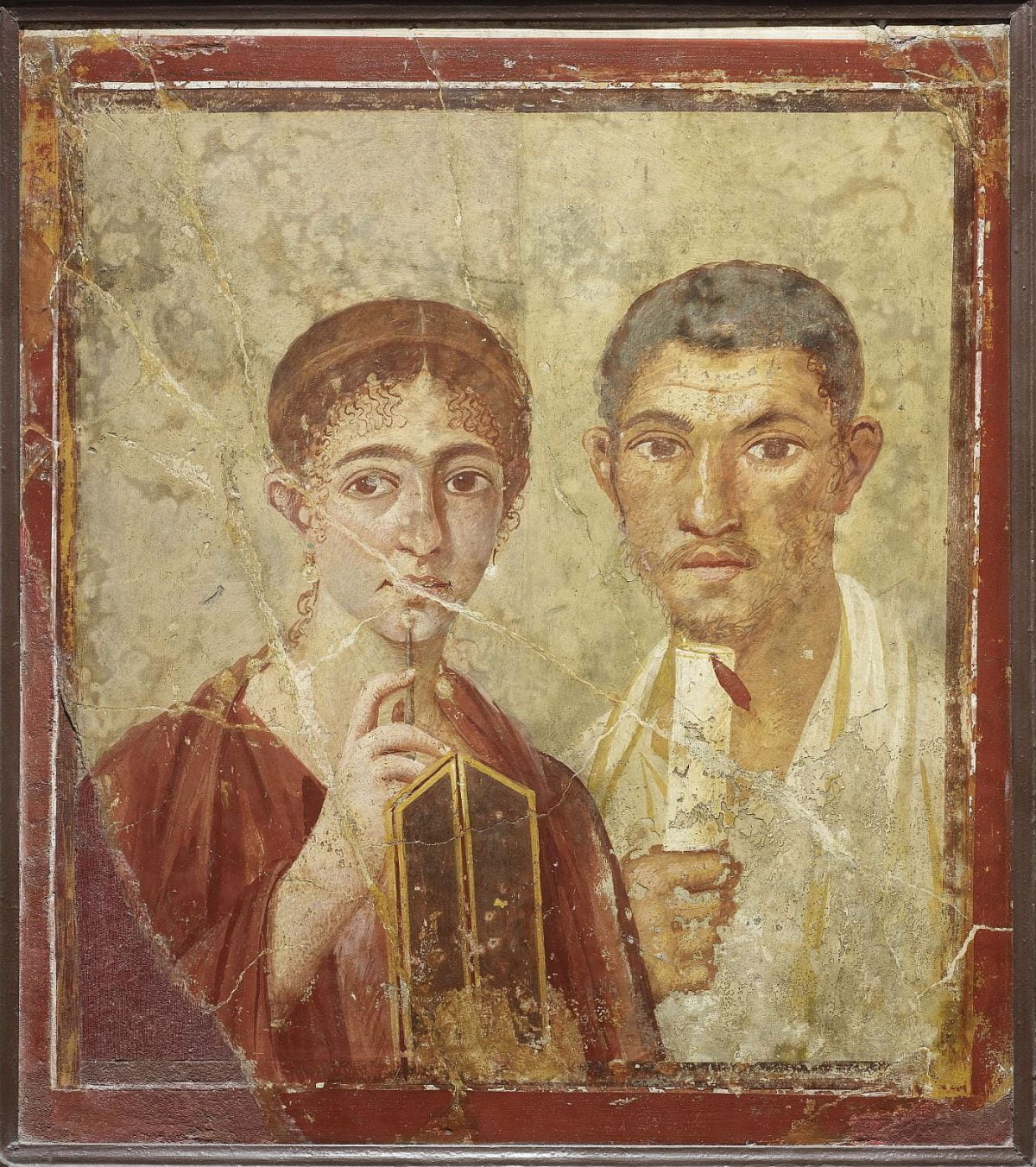A meticulously detailed painting, possibly from the 16th to 19th century, depicts a couple in formal attire. The woman, positioned on the left, has curly hair, brown eyes, thick eyebrows, and very light skin. She wears a dull red robe or dress and is holding a brown container with gold trim or possibly a thin golden object with an antenna-like feature near her chin. She gazes off to her right, which is the viewer's left. The man, on the right, has short black or brown hair, a short beard and mustache, and darker skin. He appears to be in his 20s or 30s and is dressed in a white shirt or jacket with yellow accents, holding a rolled scroll with a red feather near his chin. The background is a creamy white, and the painting itself is encased in a distressed black frame with a red border. The portrait exudes an antique charm, capturing the essence of its era through detailed facial features and attire.